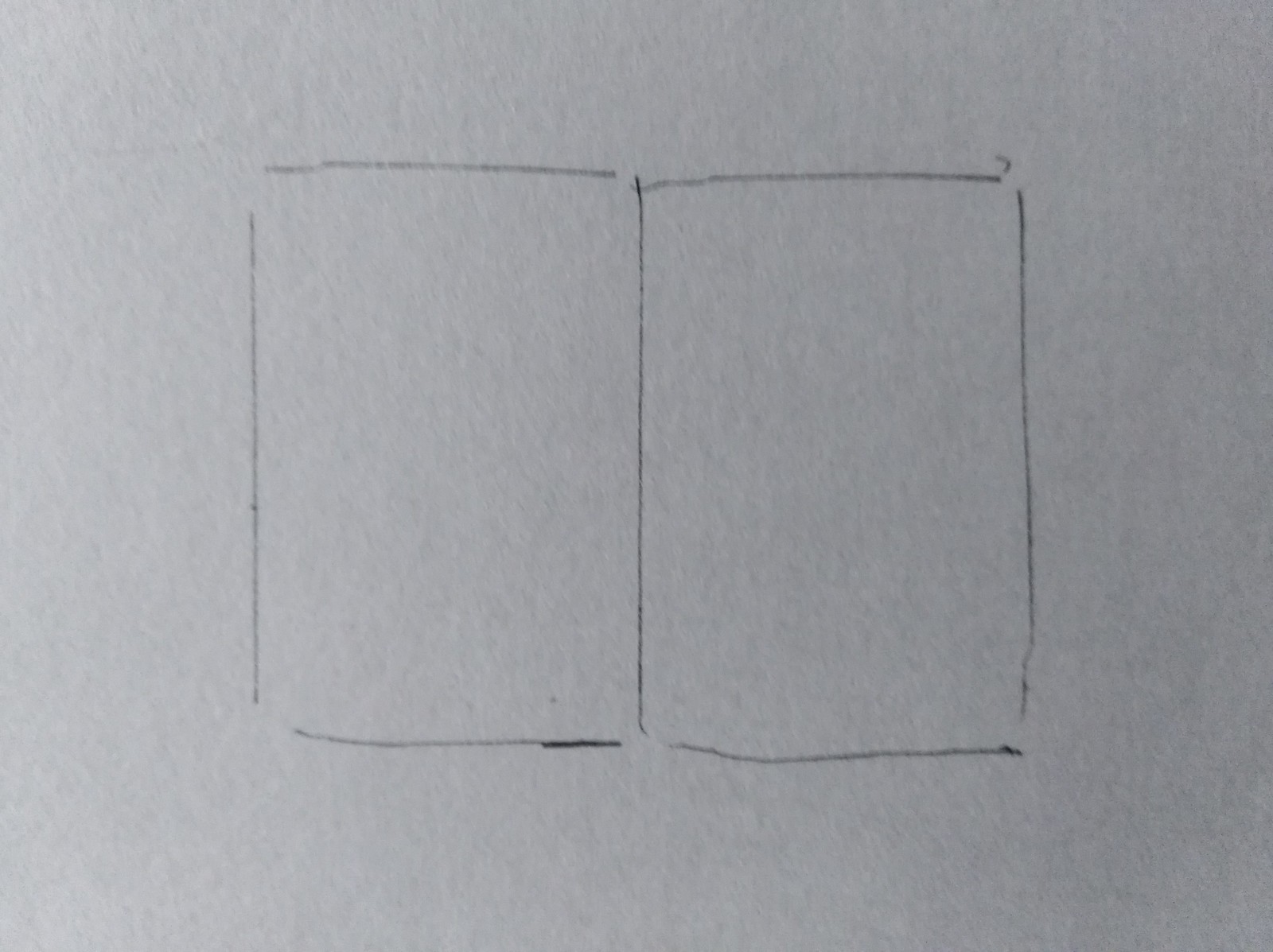The image showcases a simple yet textured piece of white paper, potentially white cardboard due to its coarser appearance. The focus of the image lies in the pencil outline of two adjacent rectangular vertical boxes, faintly reminiscent of an open book. These boxes are merely sketched with their corners somewhat disconnected, suggesting a hasty and imprecise drawing. The separation between the boxes is marked by a central vertical line. Notably, the vertical lines of the rectangles are relatively straight, possibly drawn with the aid of a ruler or book edge, whereas the top and bottom horizontal lines appear to be hand-drawn, lacking the precision of the vertical boundaries. The juxtaposition of the ruler-straightened verticals with the freehand horizontals lends a raw and unfinished character to the sketch.